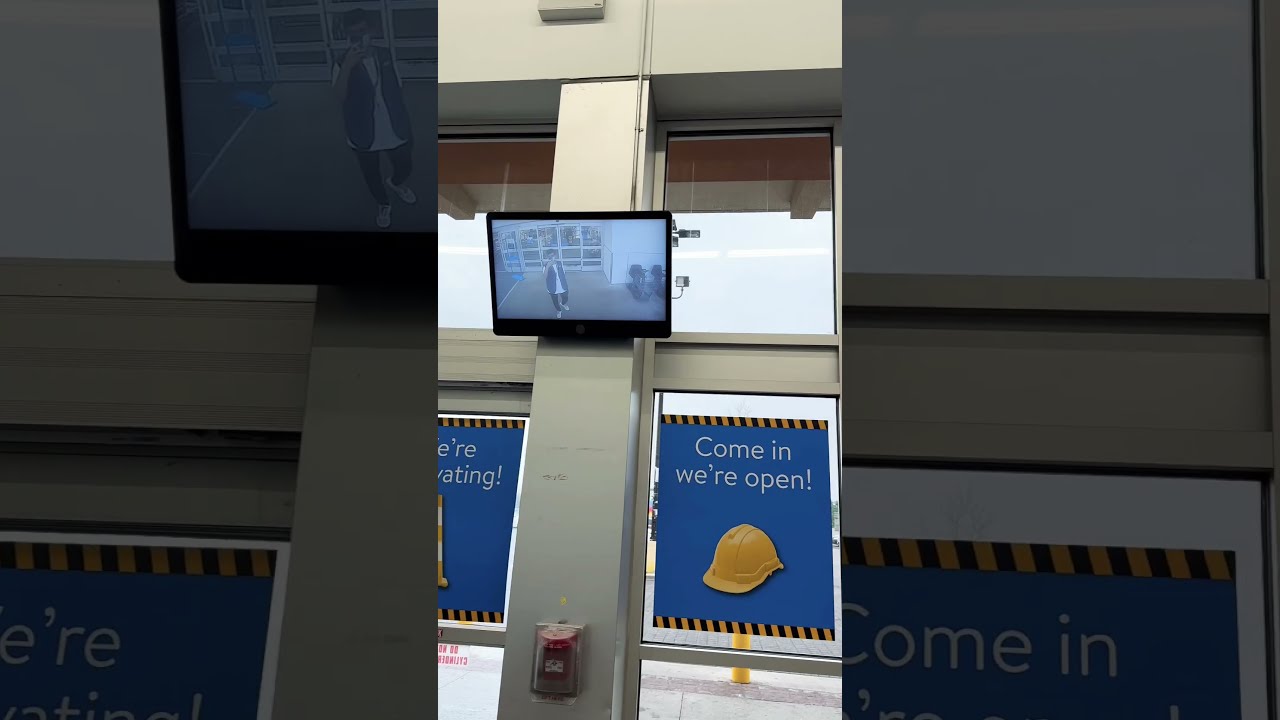The image is a surveillance camera screenshot capturing the front entrance of a store, which could possibly be a Walmart supercenter based on the blue and yellow color scheme. The vertical orientation of the screenshot shows a modern storefront featuring large sliding glass doors. Situated above the doors is a long tan beam connecting the wall to the ceiling, and attached to this beam is the surveillance camera. The store interior and exterior are visible through tall windows flanking the entrance.

In the center of the entrance, there is a person wearing a blue vest, white shirt, black pants, and a face mask, possibly acting as a greeter. The colors in the image appear somewhat diluted, yet the greeter's attire and surrounding colors of gray, black, red, and white are still discernible.

Prominently displayed on the glass doors and windows are multiple blue posters featuring the message "Come in, we're open" in white text, accompanied by an image of a yellow hard hat. These posters have black and white stripes along their top and bottom edges. Just below the surveillance camera monitor, a red encased fire alarm is visible next to the entrance. The overall setting evokes the feeling of casually stepping into a Walmart supercenter in 2024, with a modern aesthetic and essential security installations in place.